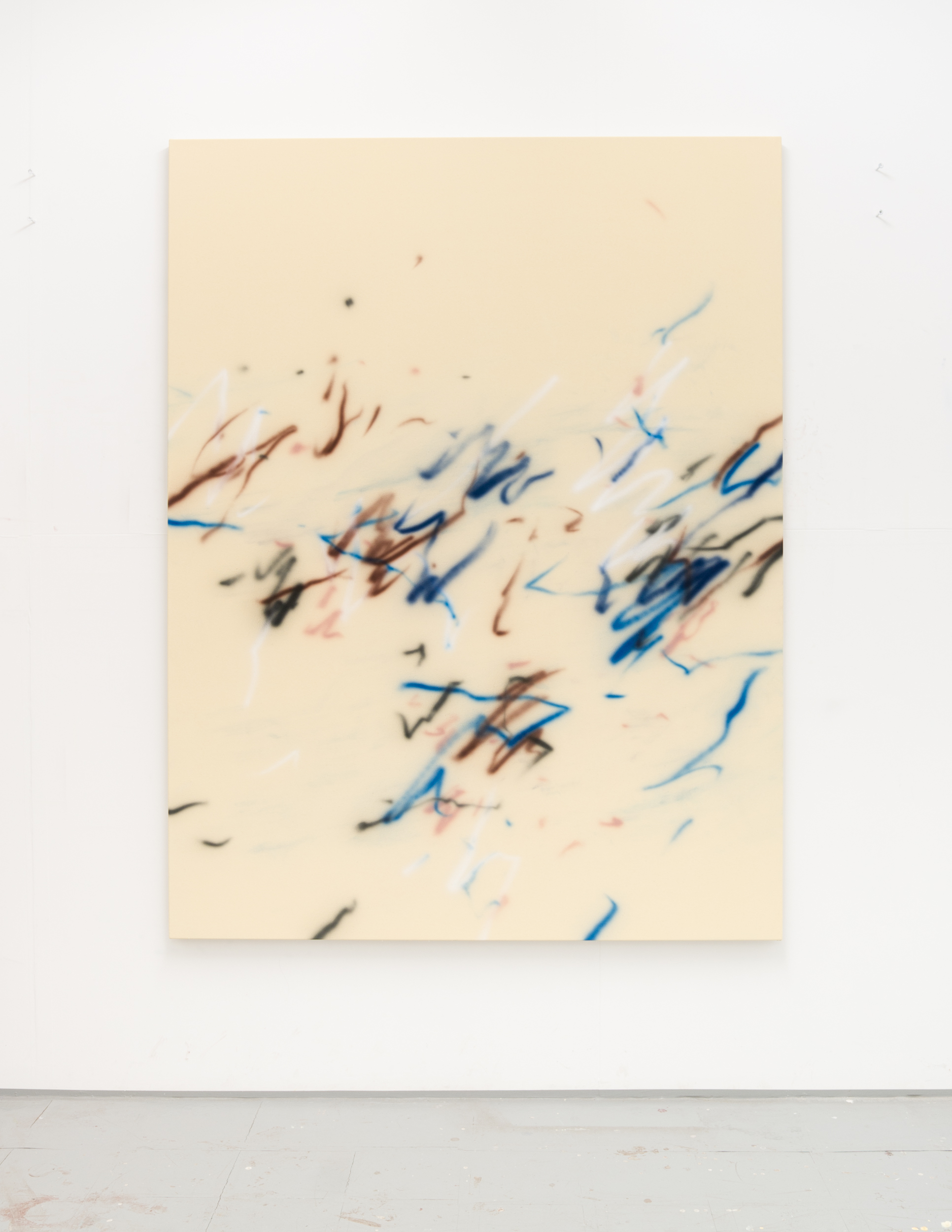The image features an indoor color photograph of an abstract painting hung on a pristine white wall, with a gray floor at the bottom. The painting itself is a large rectangle in a creamy yellow color, reminiscent of cream cheese or soap. Dominating the center of the artwork are numerous multi-colored, squiggly lines and streaks, primarily in shades of blue, brown, black, and white, with a few pink hues interspersed. These lines appear to be randomly and loosely drawn, giving a child-like, crayon scribble vibe. The majority of the squiggly and blurry lines converge towards the center of the piece, with the upper left and right corners of the painting remaining predominantly the creamy yellow background. Random black dots can also be seen occasionally amidst the colors. The overall effect is that of a modern, abstract artwork with no discernible pattern or structure, evoking a sense of spontaneous creativity.